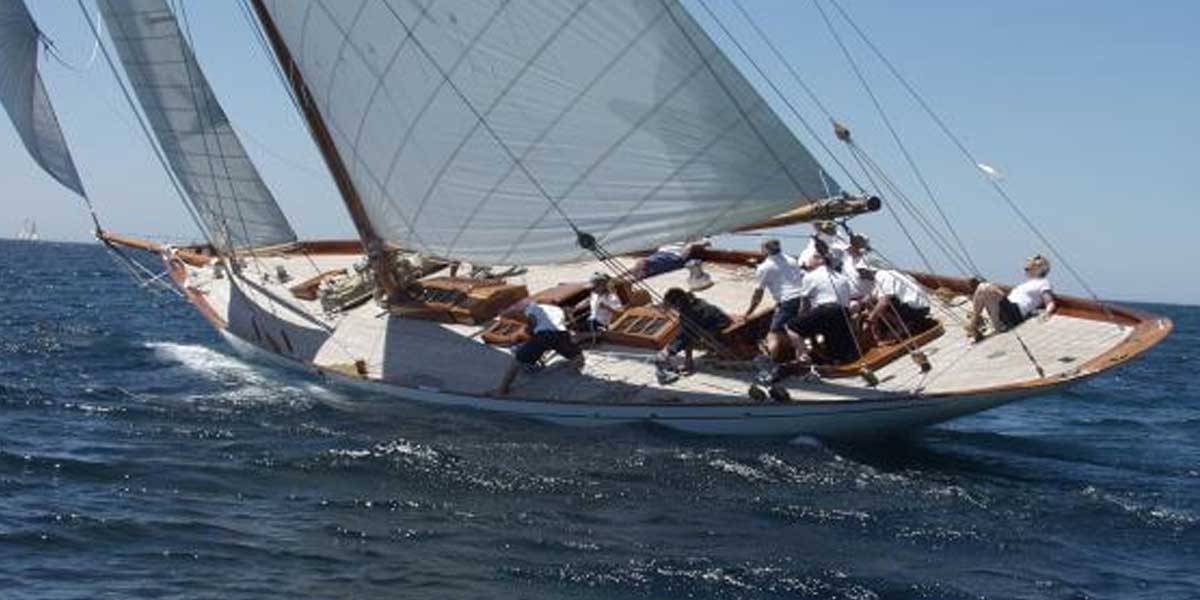The image depicts a fairly large sailboat navigating through slightly choppy, dark blue waters under a clear, cloudless sky. The sailboat, appearing cream-colored with white and brown wooden trimmings around the edges, is tilting to its right side, giving the impression that it might tip over. Seven or eight people aboard the boat are all actively engaged, wearing white t-shirts and black or navy blue shorts. One individual is precariously lying toward the back of the boat on a flat surface, while another has their foot bracing against the bottom rim, seemingly trying to stabilize the vessel. The central area of the boat, defined by brown trims, has some people emerging as if from a hollowed-out space. The boat's sails, characterized by a whitish-gray hue with diagonal stripes and visible black ropes, are fully deployed, suggesting the sailboat is moving rapidly. In the distant background to the left, another sailboat is faintly visible.